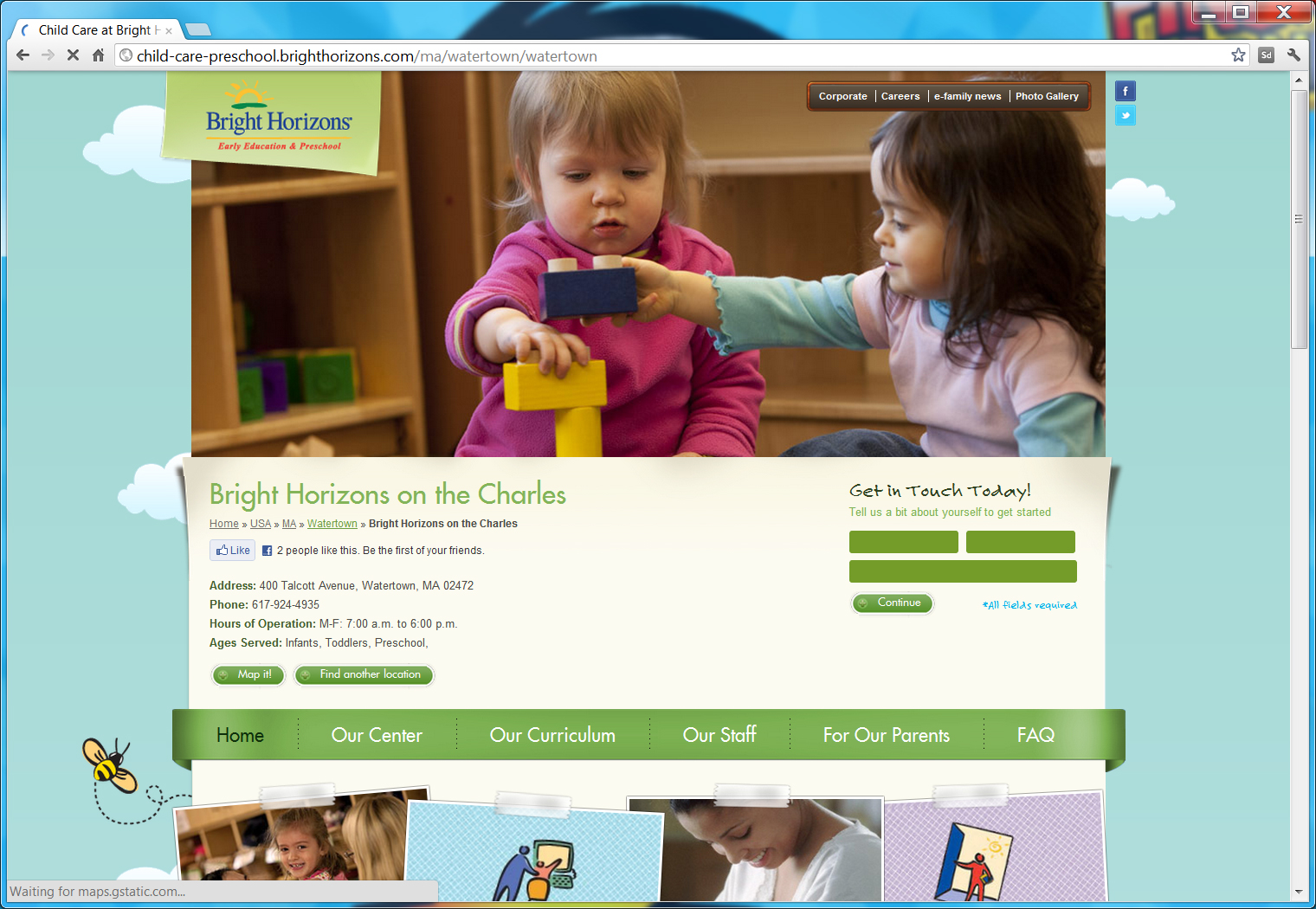The image depicts a computer screen displaying a web browser opened to the Bright Horizons Early Education and Preschool website, specifically the page for their Watertown, MA location. The URL visible in the address bar reads "child-care-preschool.brighthorizons.com/MA/Watertown/Watertown." The webpage design features an aqua background adorned with illustrations of clouds, bees, and various images.

Dominating the main panel is a photograph of two children engaged in a block-building activity. The child facing the camera has a joyful expression, while the other, seated sideways to her right, extends her hands to interlock blocks. Behind them, shelves filled with more blocks are visible, suggesting a well-equipped play area.

Below this heartwarming photograph, the site provides essential details about the center on a pale background. In green text, the heading reads "Bright Horizons on the Charles," accompanied by the center's address, phone number, hours of operation, and the age groups they serve: infants, toddlers, and preschoolers. To the right of this information is a call to action, "Get in touch today. Tell us about yourself to get started," followed by buttons to map the location or find another center.

At the bottom of the screen, there is a navigation bar. The first button on the left, labeled "Home," is in black, while subsequent buttons feature white text and read "Our Center," "Our Curriculum," "Our Staff," "For Our Parents," and "FAQ." Below this navigation bar, partially visible, are additional images related to the center.